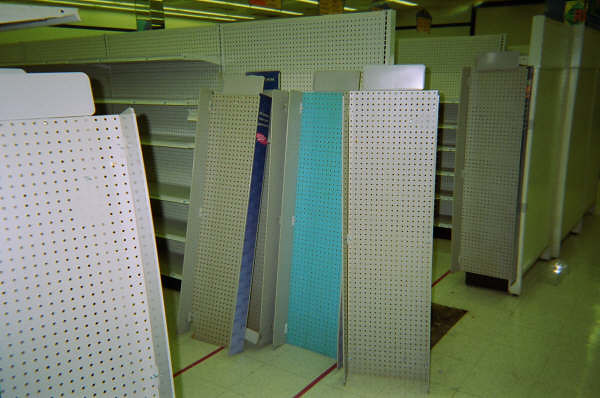The image depicts the interior of what appears to be a storehouse or a storage facility. The central focus is on a series of gray, perforated shelves mounted on a wall, which is also gray and features a pattern of small holes. Most of the shelves are gray, except for one light blue shelf in the middle and another shelf with blue edging. 

In the foreground, there is another rack that reflects light, adding some brightness to the scene. Toward the right side of the image, a white barricade is visible, contrasting with the gray tones predominant in the warehouse. The floor is laid with shiny white tiles, which reflect the overhead lighting.

In the background, several ceiling signs can be seen, though they are too distant to read clearly. The overall atmosphere is industrial and organized, with various elements contributing to the perception of a functional storage space.